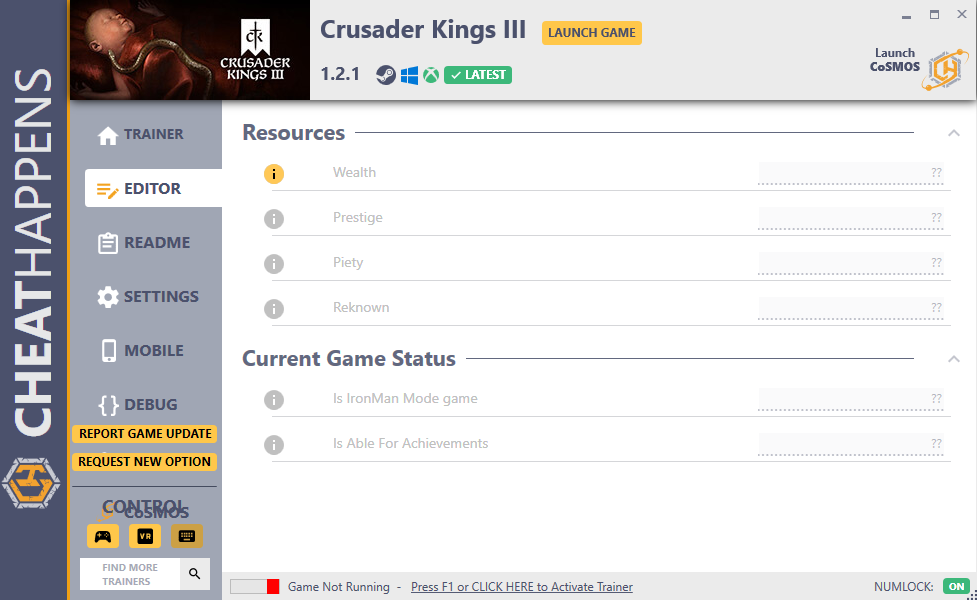Caption: This detailed screenshot captures the sleek and functional interface of a game trainer or cheat code device specifically designed for "Crusader Kings 3," developed by CheatHappens. The interface features a clean layout, beginning with the title and game image prominently displayed at the top left. Vertically aligned menu options including Trainer, Editor, Readme, Settings, Mobile, and Debug provide seamless navigation. Central to the interface is the resource section, showcasing various in-game attributes such as Wealth, Prestige, Piety, and Renown, each placeholder-marked with two question marks, indicating values to be activated during gameplay. Additionally, at the bottom, the interface includes two key options that detail the game’s status: whether it's an Iron Man mode game and if achievements are enabled.